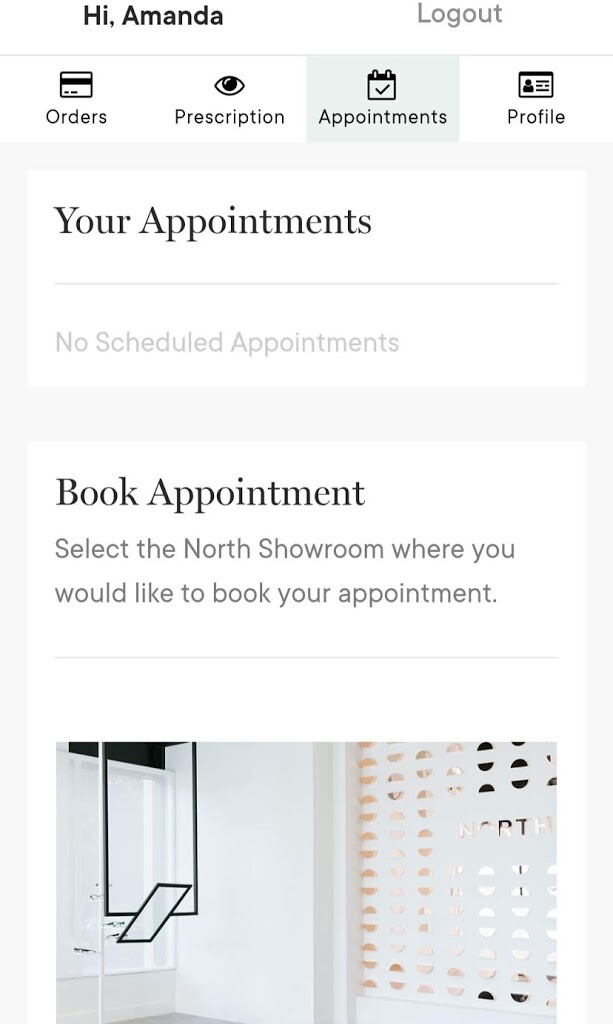The image is a screenshot from a mobile device displaying an online application for booking showroom appointments. At the top of the screen, in the upper left corner, the interface greets the user with "Hi Amanda." On the upper right corner, there is a "Log Out" button. Just below this header, there are four icons arranged horizontally, labeled "Orders," "Prescription," "Appointments," and "Profile." The "Appointments" icon is currently highlighted.

Directly under the icons, in large black text, is the word "Appointments." Beneath this, in dull gray text, the message "No scheduled appointments" is displayed, indicating that there are no upcoming appointments booked. Further down, black text instructs the user to "Book Appointments" with the prompt "Select the showroom where you would like to book your appointments."

Below these instructions, there is an image featuring the interior of a showroom with white walls. The right side of the image showcases geometric designs in the form of semi-circles, adding an artistic element to the otherwise minimalist room.